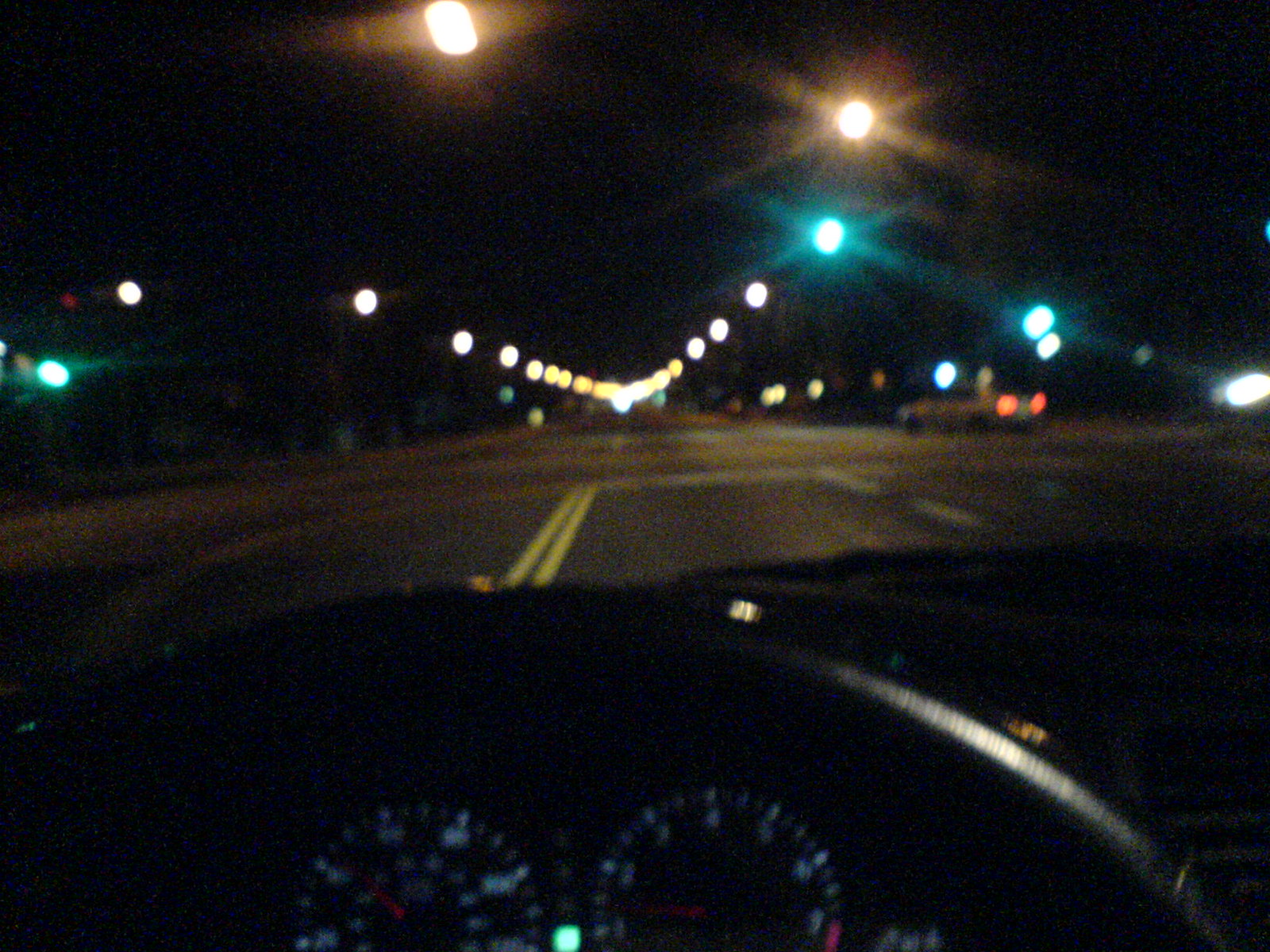A nighttime shot from behind the dashboard of a moving car, capturing a blur of illuminated dials and indicators amidst the dark interior. The city's streets ahead are dotted with numerous streetlights, casting a mix of white, yellow, and the occasional green light. A car can be seen turning right in front of the vehicle, its lights creating a glare on the steering wheel. The overall image is blurry, giving a glittering effect to the scene, with the deep black sky providing a dramatic backdrop.